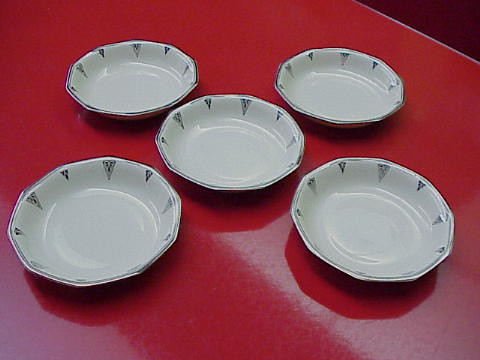The image displays five distinctive white bowls, arranged in a precise 2-1-2 formation, creating an almost star-like pattern on a big, shiny, apple-red table. Each bowl features a unique geometric design, characterized by flat-edged sides, reminiscent of rectangles, giving them a modern and slightly angular appearance. These bowls are trimmed with a dark rim, possibly black or dark gray, decorated with small, inverted triangles that extend from the rim towards the bowl's basin. The red table, smooth and reflective, dominates the picture and is bordered by what appears to be a silver band, resting against a burgundy wall evident in the upper right corner.